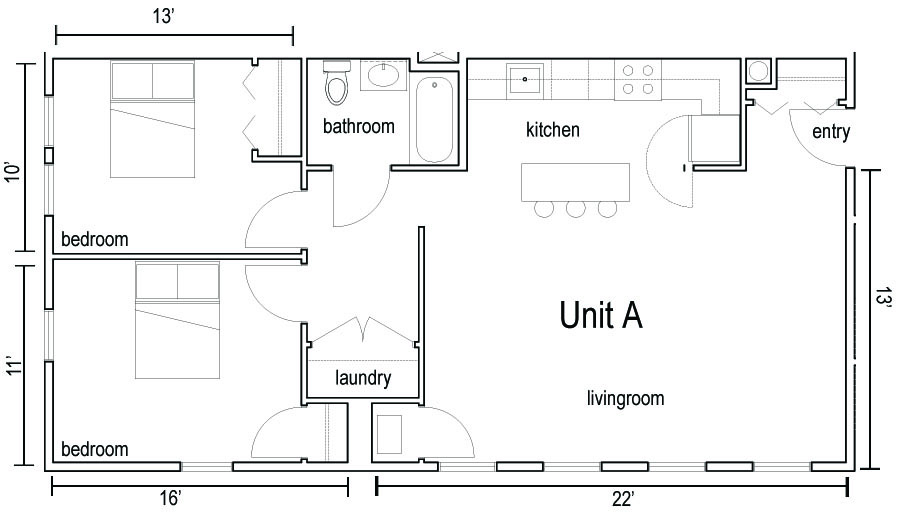This detailed architectural drawing presents a meticulously drafted floor plan of a residential house. The blueprint is characterized by prominent, dark black lines delineating the walls, with thinner lines used for windows and other structural details.

On the upper left corner of the layout, a bedroom is situated, measuring 13 feet horizontally and 10 feet vertically. This room features two windows along the left wall, a decently sized closet, and includes a double or queen-size bed.

Directly below this room, another bedroom is positioned, with dimensions of 16 feet horizontally and 11 feet vertically. It contains a smaller closet on the right side and accommodates a similarly sized bed. Both bedrooms are accessible via individual doors.

Adjacent to these rooms is a hallway leading to a compact laundry area equipped with front-facing doors. Positioned at the top left of the plan is a bathroom, complete with a full bathtub.

The drawing also highlights a spacious living room labeled "Unit A," located on the right-hand side of the house. The living room measures approximately 13 feet by 22 feet and includes a small closet at the bottom left corner. Adjoining the living room is a kitchen, equipped with a range, refrigerator, and sink, all clearly indicated in the drawing.